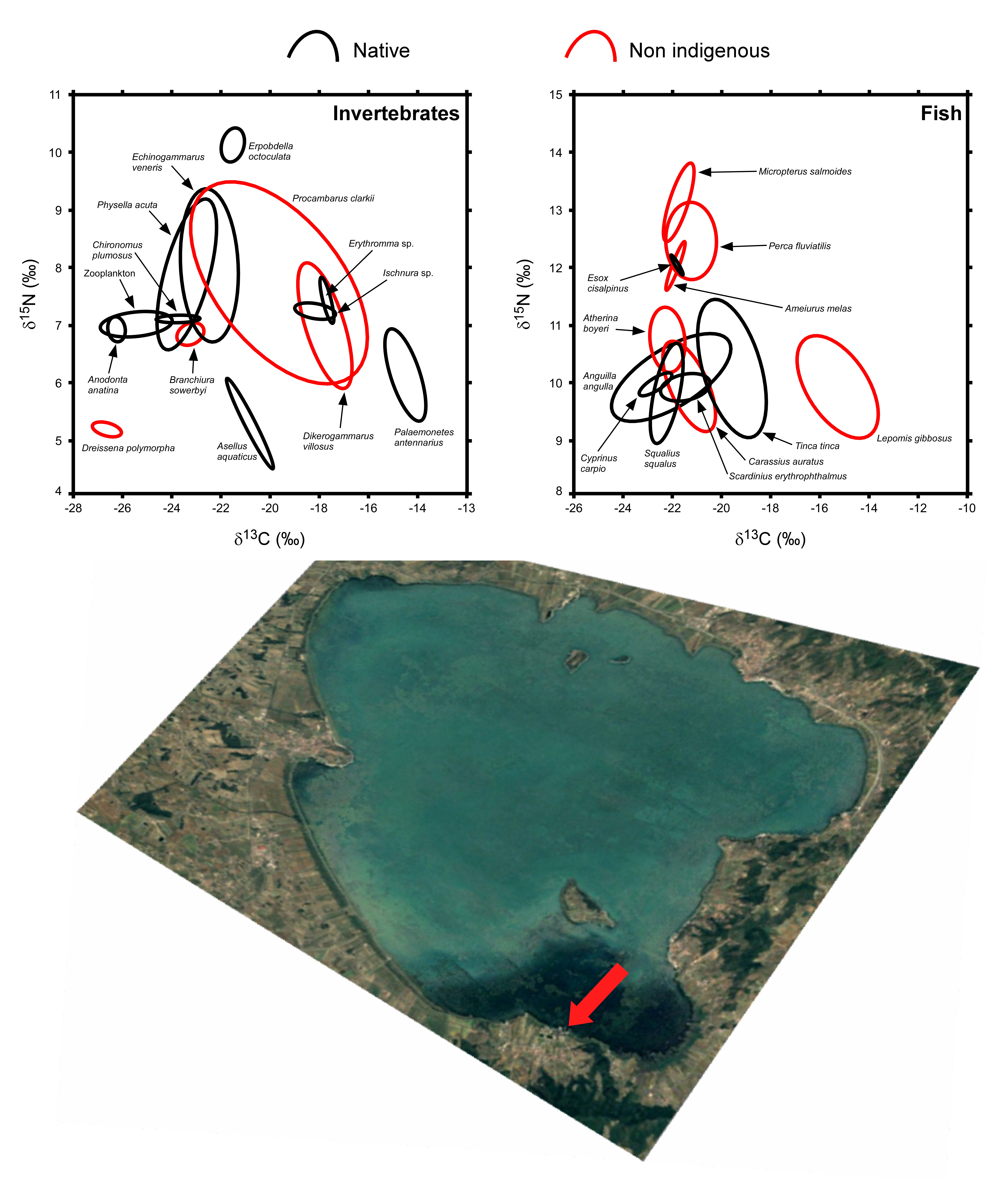The image depicts two scientific diagrams positioned above an aerial or satellite image of a large lake. The diagrams on a white background feature ovals in red and black, with the left diagram detailing invertebrates and the right one focusing on fish. Both charts have black circles indicating native species and red circles signifying non-indigenous or potentially invasive species. The left chart is labeled "native" while the right chart is marked "non-indigenous." Along the y-axis, the percentage ranges from 4 to 11, while the x-axis ranges from -28 to -13, potentially representing a nitrogen versus carbon table (Delta 15N for nitrogen and Delta 13C for carbon). Below these diagrams, the aerial image showcases a turquoise blue lake surrounded by green vegetation and farmland, with small buildings appearing as specks due to the high altitude of the image capture. There is a small island toward the bottom of the lake, docks, and a darker area of water pointed out by a red arrow, possibly indicating the sample collection site for the biological data.